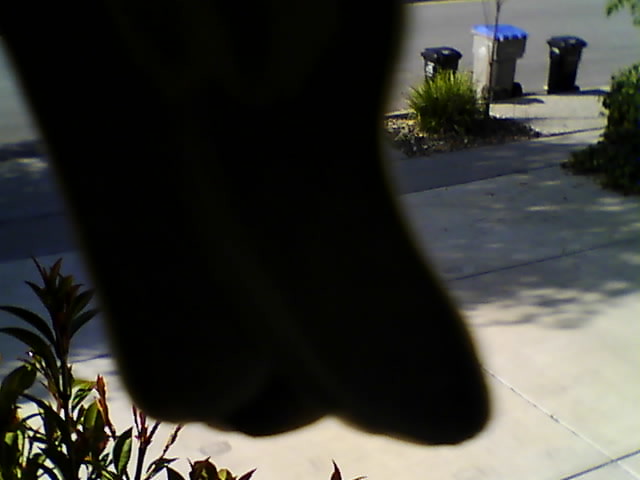This photograph captures a close-up of a security camera outside a home, partially obstructed by a large, vertical, fuzzy object with dark green and brown hues and various lobes. The object appears to be hanging down directly in front of the camera lens, obscuring the view. In the background, a wide concrete driveway leads to the curb, where three garbage cans are set out for collection. The largest trash bin is light gray with a royal blue top, flanked by two smaller black receptacles. To the left in the foreground, there is some visible foliage. Further back, near the garbage cans, a small boulevard with a tree and a flower bed containing a bush and landscaping stones is visible. Additional foliage is seen in another corner of the image. The scene is bathed in sunlight, with tree shadows cast onto the pavement, suggesting a bright, clear day.